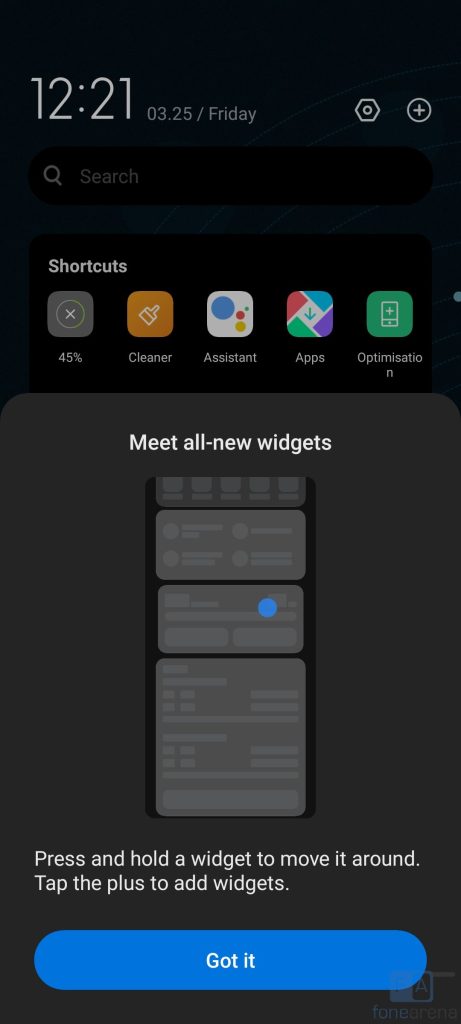The image displays a portion of a smartphone interface, rich in detail and information. In the upper left-hand corner, the time is prominently shown as "12:21" in large white numerals, while directly beneath it, the date "03-25" and the day "Friday" are displayed in a subtler gray font. 

In the upper right-hand corner, a small hexagon symbol containing a small circle is visible, accompanied by a circular plus sign. Below these icons, a magnifying glass and a search bar labeled "search" encourage user interaction.

Further down, a row of five shortcuts is arranged from left to right. The first shortcut features an "X" symbol within a circle, indicating "45%". Next is a brush icon labeled "Cleaner", followed by circular shapes representing "Assistant". The fourth shortcut displays diamonds with a downward-pointing arrow, denoted "Apps". The final shortcut shows a rectangle with a plus and minus sign inside, labeled "Optimization".

Below these shortcuts is an instructional section titled "Meet all new widgets". It advises users to "press and hold a widget to move it around" and "tap the plus to add widgets". A conspicuous blue oval button labeled "Got it" offers an acknowledgment option.

Finally, the faint text "Phone Arena" is subtly placed in the bottom right-hand corner, marking the source or context of the image.